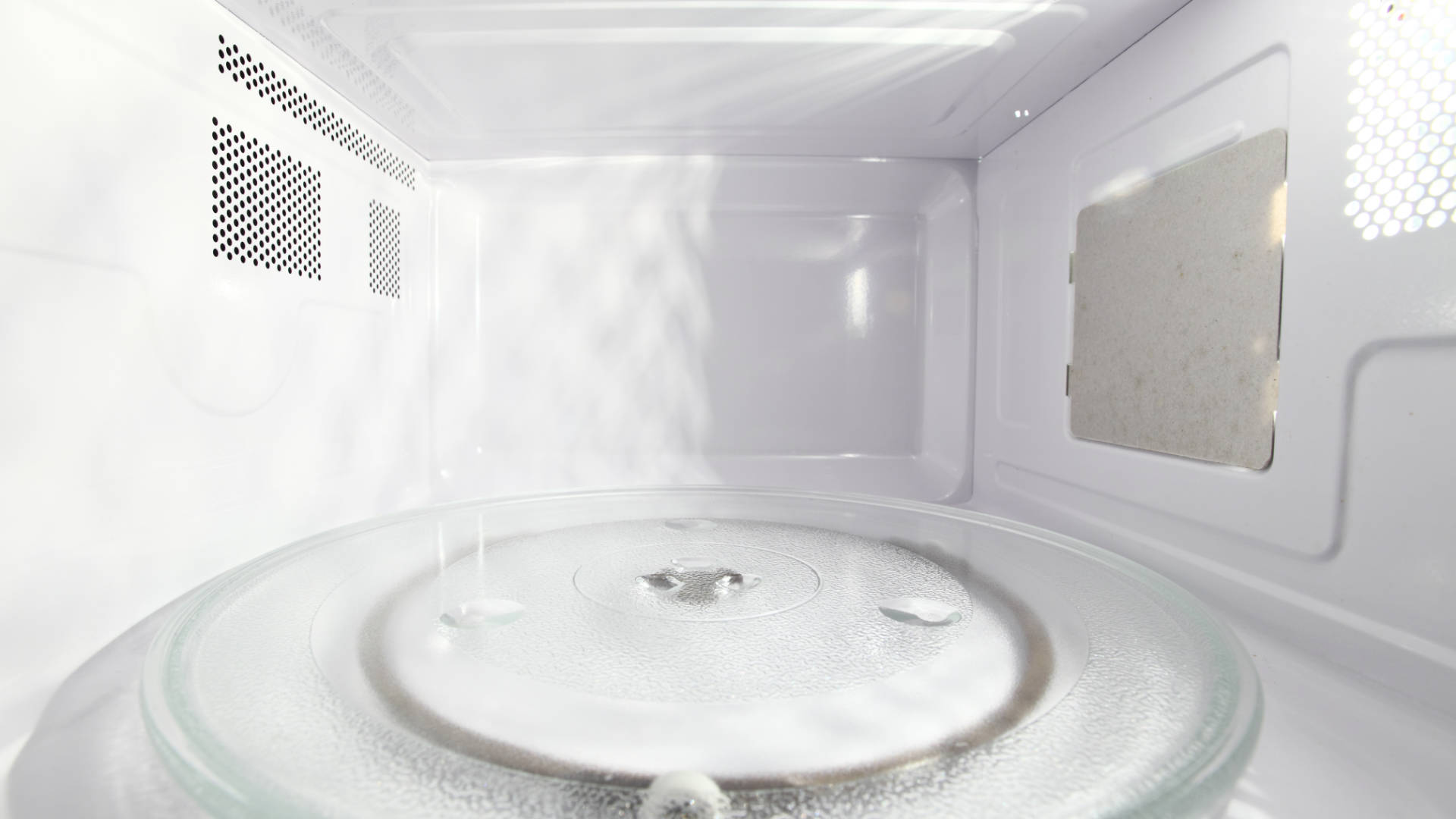The photograph is a detailed capture of the inside of an immaculately clean microwave oven, predominantly white. The spacious interior showcases a transparent glass rotating dish positioned at the bottom. This dish features a central divot with four surrounding divots arranged in a cross pattern, encircled by a darker ring. The walls and the ceiling are a plain, uninterrupted white metal.

Distinct to the left-hand side, there are several ventilation grates. These include a long horizontal rectangle at the top, followed by three progressively smaller and square-patterned grates underneath. On the right-hand side, there's a noticeable metal panel affixed to the otherwise white interior wall, alongside a small honeycomb-shaped pattern. Adding to the details, the top right corner houses another grid of circular holes that shield a light source, likely a bulb. The entire scene is well-lit and shadowed minimally, a result of the open microwave door which casts a faint shadow at the back.